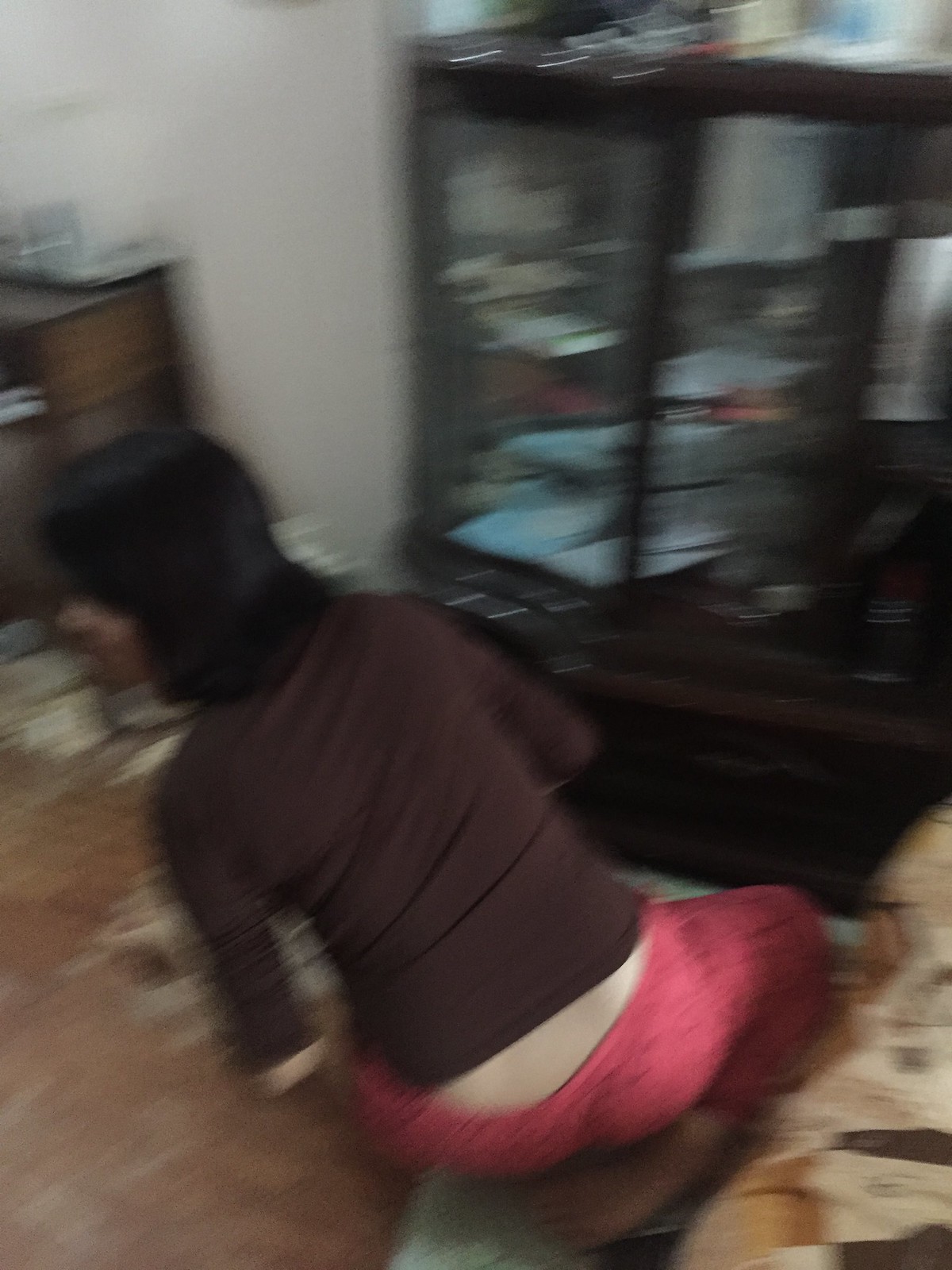This image is notably blurry and of low resolution, making details difficult to discern clearly. However, the central subject appears to be a person positioned in the middle of the scene. The person is facing away from the camera, with their head slightly tilted to the left. They have black hair and are dressed in a brown top paired with pink pants. The individual seems to be in a seated posture. In front of them is a piece of black furniture, which includes a see-through section with doors at the top. The image is cluttered with various items, adding to the overall busyness of the scene.